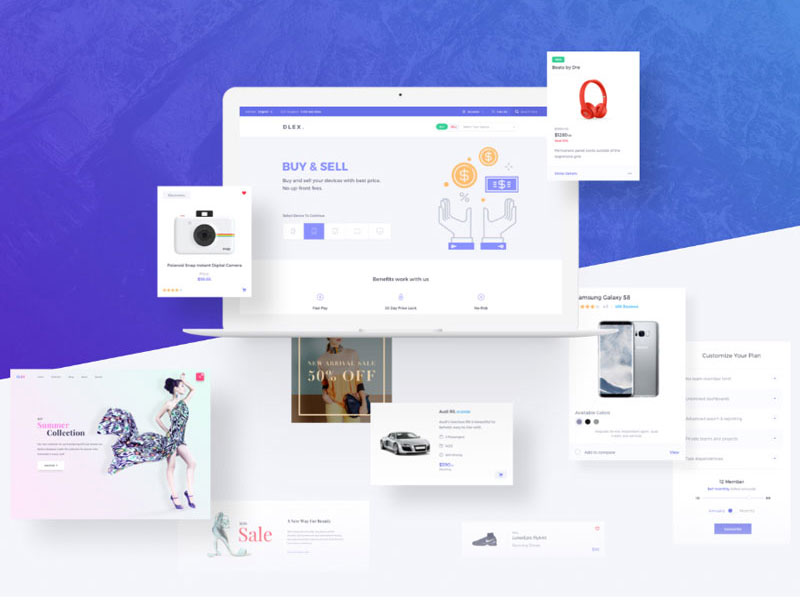The image appears to capture the background of a computer screen, filled with various images and textual elements that are somewhat blurry, making full comprehension challenging. 

At the top of the screen, there's a medium blue background hosting a few photos. The leftmost image is a photograph of a camera. Though much of the text on this photograph is indistinct, the words "digital camera" can be discerned beneath the camera picture. In the top right corner of this photo, a red heart symbol is visible.

To the right of the camera photo is a much larger image that resembles a web page, featuring the partially readable text "buy and sell" and "Buy and sell your...," with the remaining text being too blurry to decipher. On the right side of this web page, there is an illustration of two hands with dollar signs and a percentage sign floating above them, alongside a blue paper marked with dollar signs.

Following this to the right is an image titled "Beats by Dre" in very faint text, showing a pair of red headphones. The description below this heading is unreadable due to the blur.

The lower section of the screen includes an image positioned on the far left, showing a woman in a dress with the text "summer collection" and some other unclear text. In the center is an image featuring the text "50% off" overlaying a picture of a person modeling an outfit. Below this is a photograph of a sedan with the word "Audi" visible, though the accompanying text is too blurry to interpret completely.